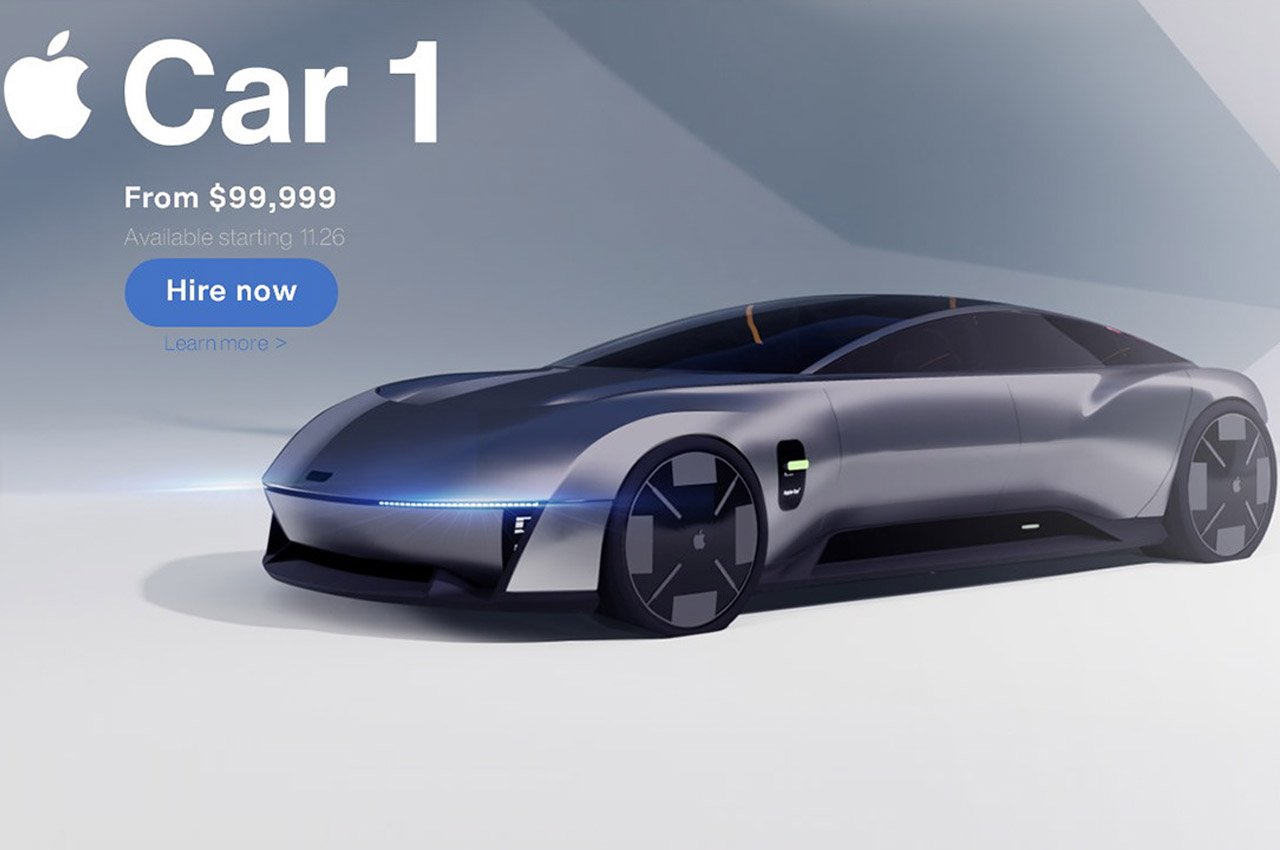This image is a highly detailed 3D color rendering, showcasing a futuristic, silver concept car from Apple, aptly named "Car 1". The car, with its low-lying, aerodynamic design, features a distinctly rounded top and flat base. The sleek vehicle, lacking visible entry handles, showcases unconventional black tires with gray slots and flared fenders surrounding the front wheels. The headlights are subtly integrated, almost invisible, blending seamlessly with the vehicle’s smooth design. The car's front hood faces left, with its rear directed to the right, positioned mere inches above the pristine white ground. 

A grayish backdrop in varying shades sets the stage, displaying a white Apple logo at the top left corner. Adjacent to the logo, bold white text reads "Car 1", followed by the price "From $99,999" in smaller white print. Below, faint white text announces its availability starting 11-26. A blue button beneath these details carries the call to action "Hire Now Inside" in white, and underneath, faint blue text invites viewers to "Learn More". This image masterfully combines 3D illustration with graphic design elements, encapsulating the allure of a next-generation automotive concept.